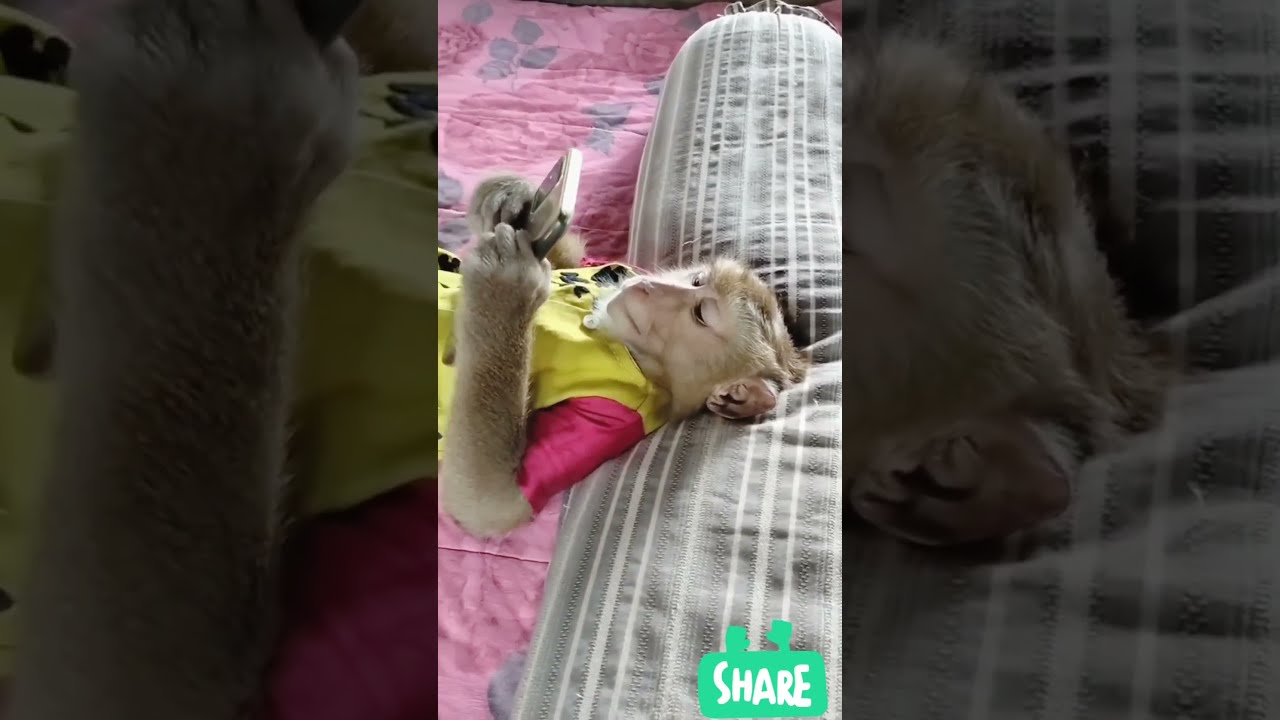In this charming and amusing vertical image, we see a light brown rhesus monkey sprawled comfortably on a pink floral blanket. The monkey's head rests on a long, tube-like body pillow adorned with gray and white stripes running the length of it. Dressed in a vibrant yellow shirt with pink sleeves that end just above his elbows, the monkey's furry arms and expressive face are fully visible. He holds a cell phone in both hands, gazing intently at the screen, mimicking a human lounging in bed. The photo is presented in three panels: the center panel showcases the full scene, while the outer panels zoom in on the adorable details, emphasizing the cuteness and human-like behavior of the monkey enjoying his electronic device.